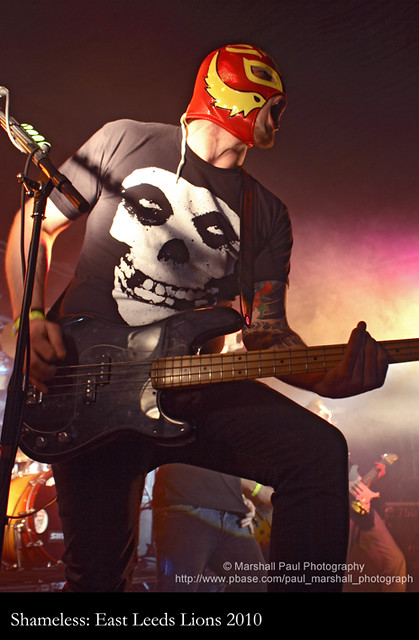In this atmospheric nighttime concert image, a striking frontman dominates the stage, wearing a vibrant red and yellow wrestling mask that covers his entire face, with eye and mouth slots and trailing white strings. He's clad in a black t-shirt featuring a white skull graphic, partially obscured but noticeably staring upwards. Playing an all-black electric guitar, he stands with his mouth wide open, possibly singing or screaming, and his right arm adorned with bracelets and tattoos. Behind him, hazy smoke and stage lights create a dramatic backdrop where a drummer and another guitarist are visible. The bottom of the photo is marked by a black rectangle with white text, reading "Shameless East Leeds Lions 2010," while "Marshall Paul Photography" and the photographer's website are noted to the side.